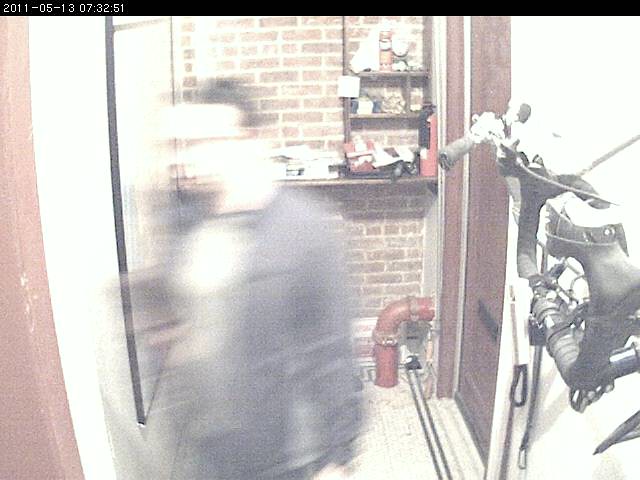The image, likely captured by a security camera, displays a blurred figure of a man in motion, suggesting low image quality and potential night vision. The man has short black or dark brown hair and possibly some facial hair. He is wearing a dark gray, dark blue, or black shirt featuring a lighter-colored logo resembling a mushroom cloud with a base. The scene appears to be in a basement, garage, or utility room characterized by a white tiled floor with black lines and decorations. Notable details include a dark wood door and a nearby dark-colored bicycle or motorcycle, with possible parts scattered around. The background boasts a brick wall with a hanging shelf or bookcase made of dark wood, displaying indistinct tchotchkes. To the bottom left, an L-shaped red pipe emerges from the floor. A hallway extends into the left of the image, with another entryway visible, indicating the man may have entered through the door on the right. The general ambiance of the area is dim, enhancing the sense of motion and blurred features.